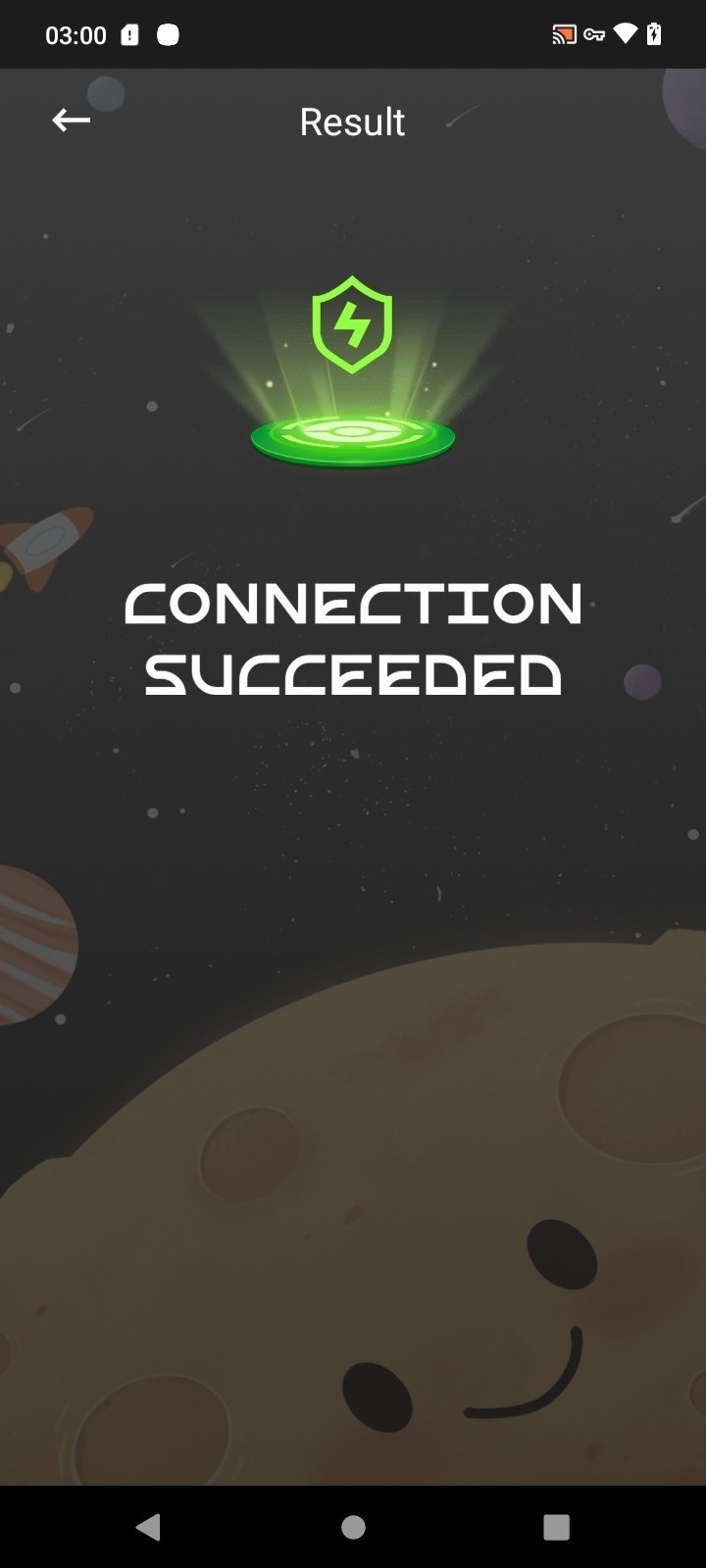This screenshot captures a webpage with a dark-themed background, predominantly featuring shades of black and gray. At the top of the page, there is a sleek black bar containing several white elements: starting from the left, it shows "03:00," followed by a square icon with a missing corner suggesting an option or symbol, a comment section, a sound icon, a battery charge indicator, a key icon, and a lock symbol.

The main section of the page features a darker gray background adorned with lighter gray dots, reminiscent of stars or planets scattered across a night sky. Dominating the bottom third of the page is a pale, creamy yellow sphere resembling a planet or a moon, complete with darker yellow crater markings and two black spots connected by a slash, forming a simplistic smiling face. The craters have edges that rise slightly, adding depth to the depiction. 

To the left of this yellow sphere, there is a partially visible orb with white and red stripes, modest in size and brightness. Rising above, about two-thirds up on the left side of the page, a white rocket with a red tip and red fins is positioned.

At the top center of the page, the word "Result" is prominently displayed, with only the "R" capitalized. To the left of this text, there's a left-facing arrow. Positioned below the word "Result" is a green circle emanating yellow and green light, which has a celestial or UFO-like appearance due to its radiating stars. At the center of the green circle is a semi-transparent shield icon with a lightning bolt, blending green and gray hues. Completing the scene, bold white capitalized text at the bottom declares "CONNECTION SUCCEEDED," confirming a successful interaction or status on the page.